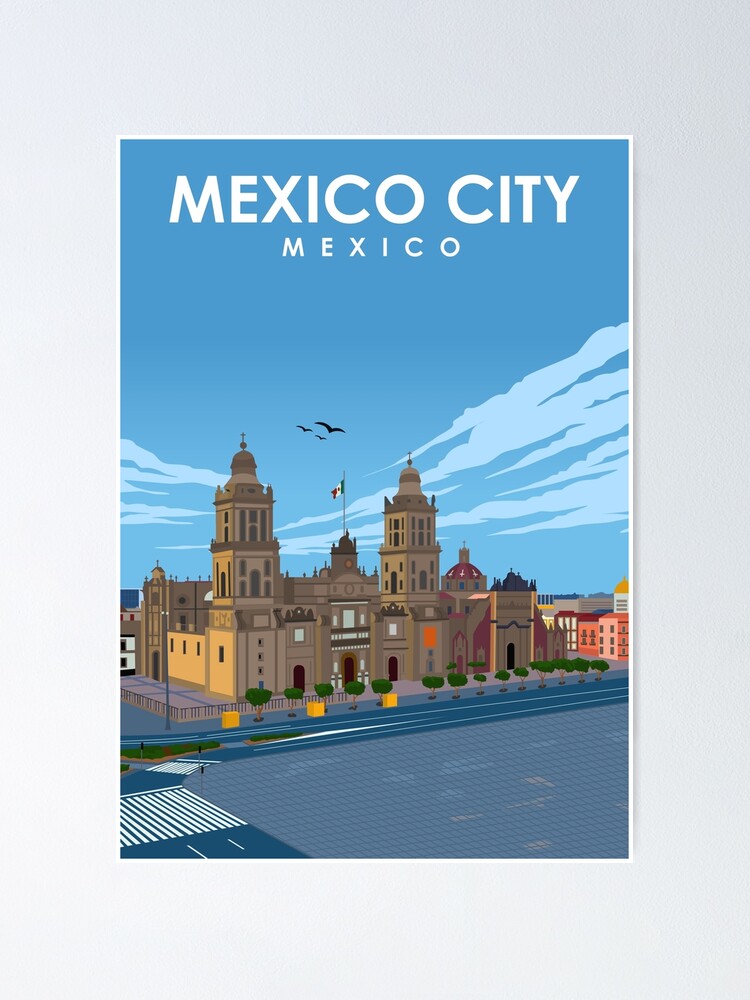The image is a detailed illustration, resembling a painting, of a prominent landmark in Mexico City, Mexico. This landmark appears to be a grand government building or a palace, with distinctive brown architecture featuring dome-shaped structures, tall towers, and large entrances. The dome has a Mexican flag atop it, with red, green, and white colors. Surrounding the landmark are neatly arranged trees and a barricade. The background depicts a blue sky with light clouds, while some buildings behind the main landmark show hints of pink among other colors.

In the foreground, there’s a prominently blue paved walkway and a four-lane road, divided by a planted divider with white markings and additional plants. Light posts and electric poles line the roads, which connect to the city center. This focal scene is framed by a gray border and the entire composition is titled "Mexico City, Mexico" in bold white uppercase letters at the top.